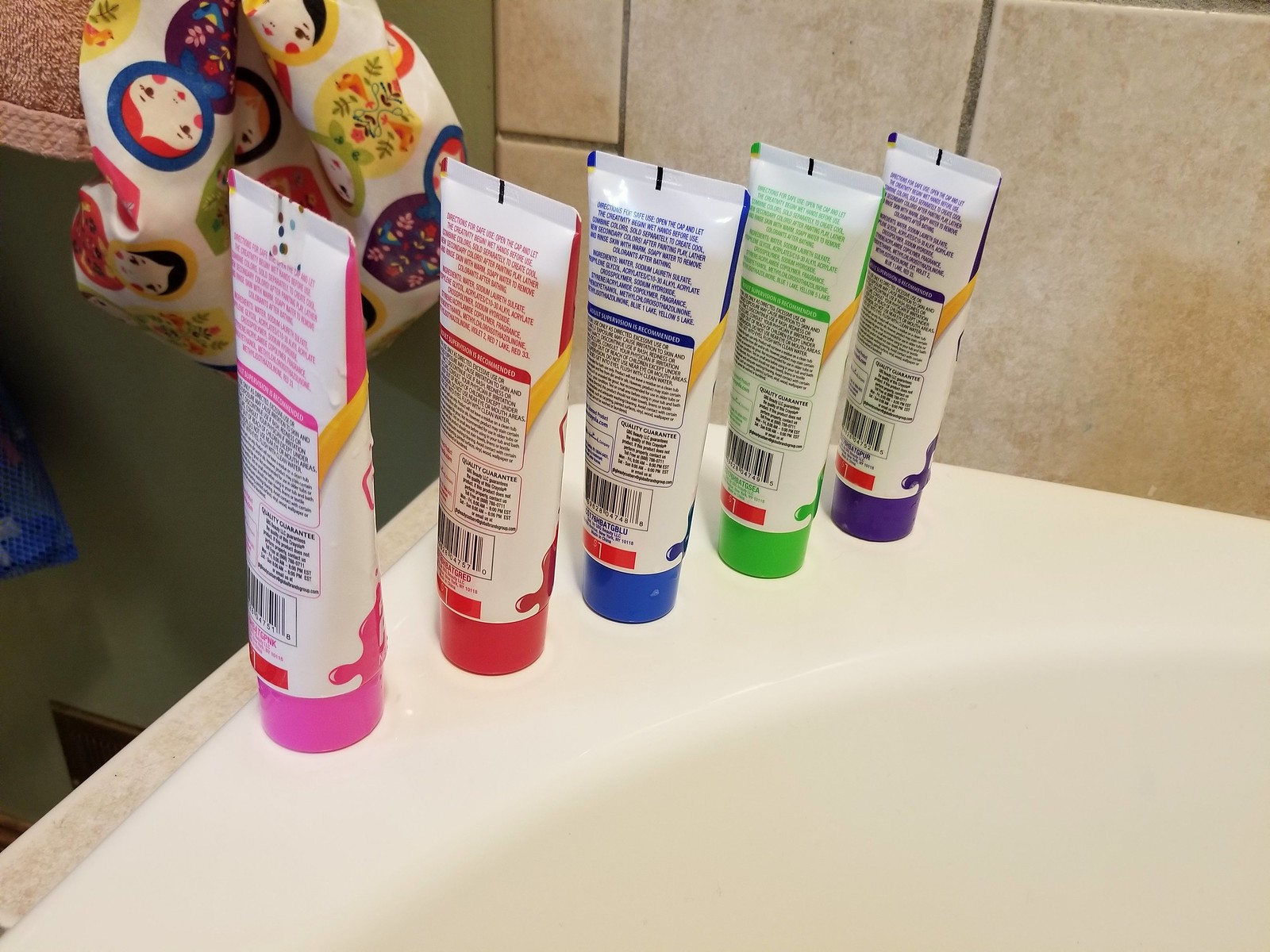This detailed photograph captures a colorful, organized scene on the rim of a white porcelain bathtub in what appears to be a bathroom. The bathtub is placed against a backdrop of tan tiles with a slightly darker grout, complemented by a green wall to the left. Five plastic tubes are neatly aligned, each standing on its cap, which creates a stable base for them. From left to right, the caps are pink, red, blue, green, and purple, with corresponding matching text on the back of each tube, though the writing is too small to read. The tubes are likely containers for temporary hair dye or finger paint soap for children, given their playful, vibrant colors. Adding to the bathroom's character, a colorful towel decorated with Russian nesting dolls and another brown towel are visible in the upper left corner, and a multicolored shower cap with Little Red Riding Hood characters hangs from a hook on the wall. The overall setting evokes a lively, child-friendly atmosphere.